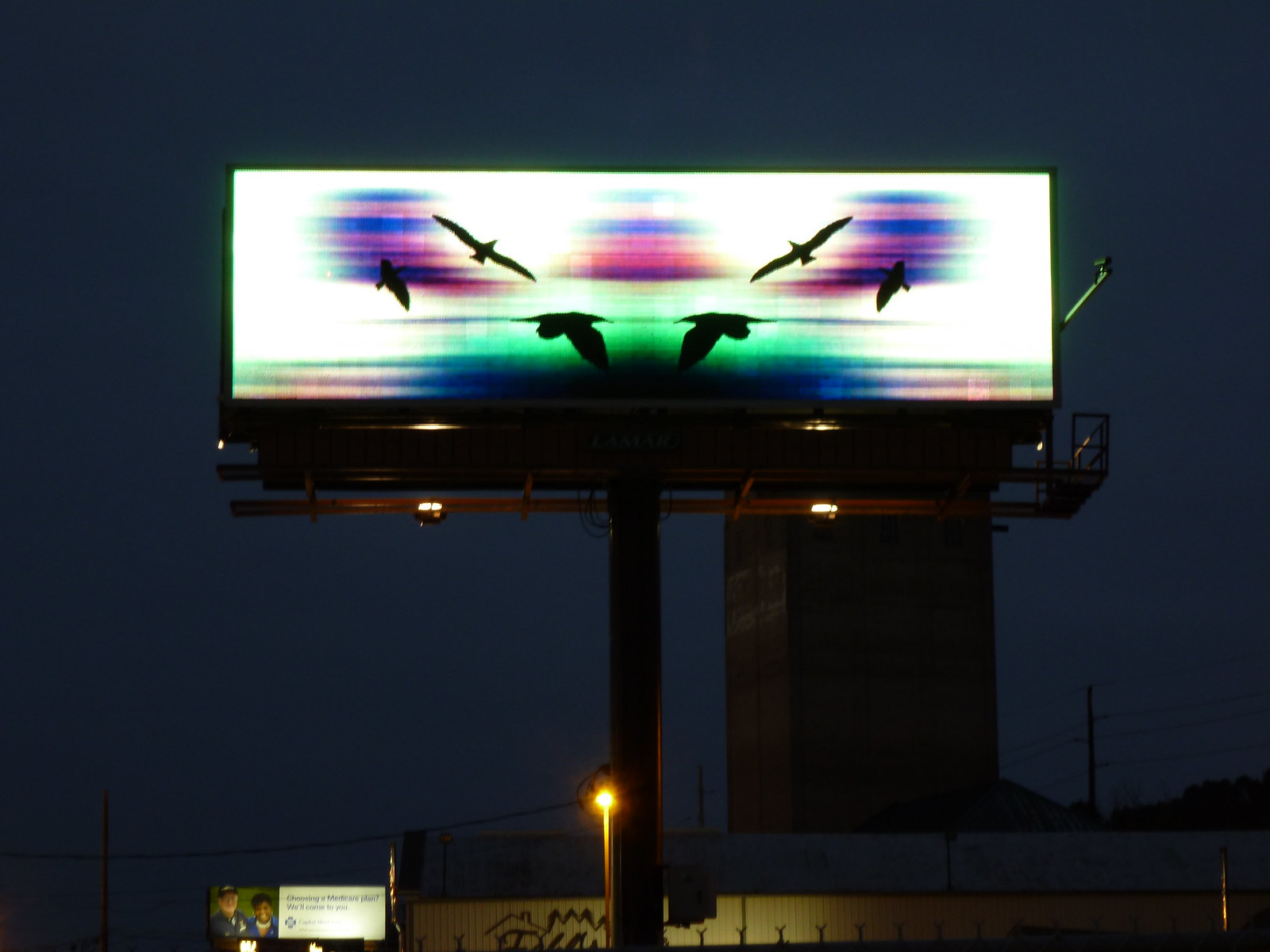The photograph, taken at night, features a wide image with a digital billboard dominating the center. The billboard, which is roughly 3-4 times as wide as it is tall, displays a vibrant mirrored design. Against a dark night sky, six silhouetted birds create a circular motion across the screen, flying in various directions. The background of the billboard showcases colorful tie-dye-like streaks forming distinct shapes: two crescent moons in blue and pink facing each other, a centered triangle matching the blue and pink hues, and a horizontal gradient oval transitioning from green to blue. Below the main scene, in the lower part of the image, a tan male with a white beard and a dark-skinned woman with a white necklace appear next to text related to a Medicare plan. Additionally, a building with black graffiti and an adjacent red structure are partially visible, adding depth to the nighttime setting. The digital nature of the billboard suggests that the displayed image can change, contributing to the dynamic feel of the photo.